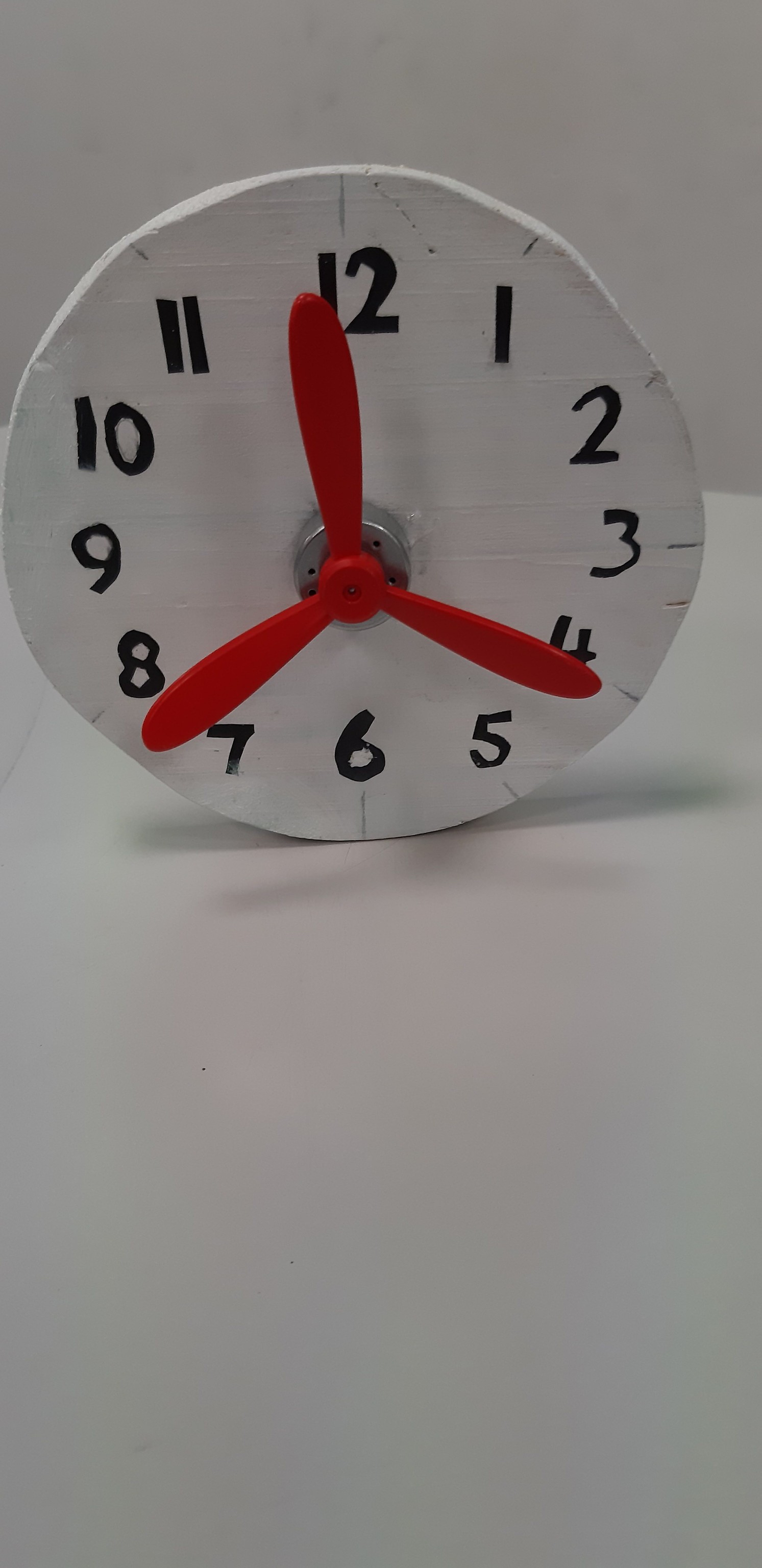This image features a unique, artistic clock crafted from a wooden piece that has been painted white. The clock face is adorned with black, hand-painted numbers marking each hour from one to twelve. The clock hands are fashioned into a three-pronged, red plastic propeller, with one hand pointing just before 12, another at 4, and the last one between 7 and 8. This creative clock stands prominently on a white table, set against a white wall in the background, giving it a minimalist and modern aesthetic. The artwork exudes a handmade, whimsical charm, reflecting the fusion of functionality and creative expression.